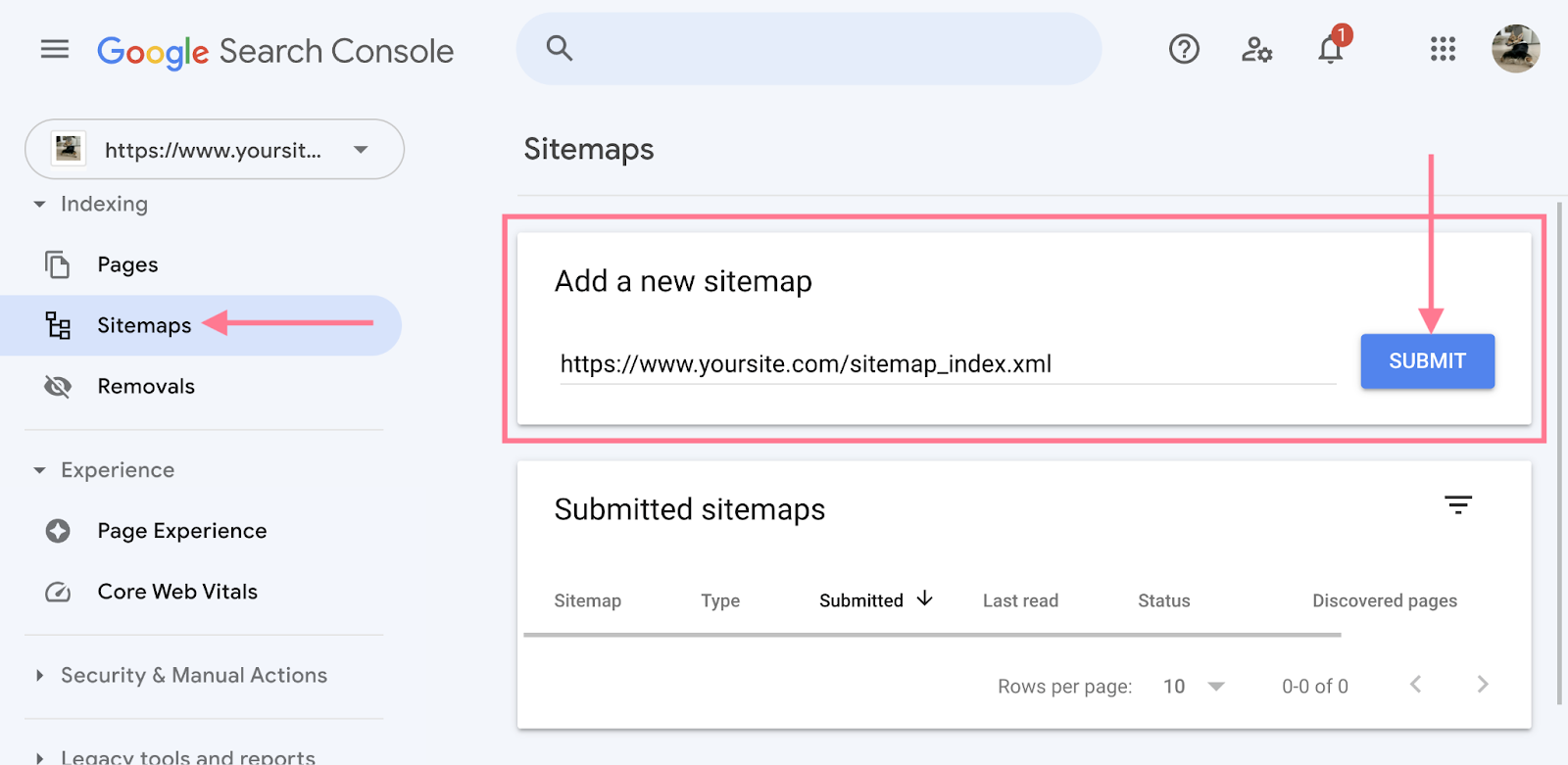The image displays a screenshot taken from a user's Google Search Console interface. At the top of the page, a search bar is visible, accompanied by a question mark icon encased in a circle for help or additional information. Adjacent to this, a silhouette of a human with a plus sign, indicative of user management options, is present. A notification bell shows an alert with the number one highlighted in a red circle, suggesting a pending notification. To the far right, the user's profile picture featuring their dog is displayed in the profile section.

On the left panel, a navigational menu can be seen. This menu includes several clickable options: an HTTPS link, indexing information, pages, sitemaps, and removals. Below a faint gray divider line, options for experience, page experience, and core web vitals are listed, each paired with corresponding icons. Further down, another faint gray line precedes sections labeled "Security and Manual Actions" and "Legacy Tools and Reports."

In the center of the interface, directly beneath the "Sitemaps" header, there is a prominent red rectangle button labeled "Add a new sitemap." Next to it, an input field for an HTTPS website is provided, alongside a submission button in blue. A red arrow directs attention downward towards the submit button, clearly indicating where user action is required.